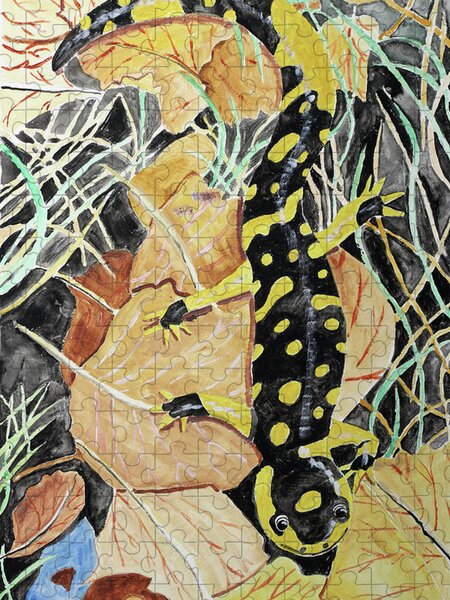This image showcases a completed jigsaw puzzle featuring a cartoonish lizard, most likely a salamander or gecko, depicted in vivid detail. The lizard, oriented vertically with its tail at the top and head at the bottom, is predominantly black adorned with vibrant yellow splotches. Notably, its body exhibits intricate patterns, including black spots and markings near its toes, while a prominent yellow dot graces its face, complemented by a wide yellow mark resembling a smile. The lizard’s eyes are cartoonishly black with white highlights, and it has two distinct black nostrils.

The background of the puzzle is a fascinating blend of alien-like, abstract elements. It comprises a mix of colors and textures, including a dark backdrop with swirling blue and yellow tendrils. The lizard appears to stand on an amalgamation of autumnal leaves and abstract floral designs—green, peach, yellow, orange, and an azure blue petal—creating an otherworldly scene. Details such as a clear outline of puzzle pieces on a flower petal and a prominently folded yellow area on the bottom right, resembling another flower, add complexity to the setting.

Overall, the cropped nature of the image, which abruptly cuts off the outer edges of the puzzle, frames the lizard and its environment in a close-up view that emphasizes the intricate design and vibrant coloration of both the creature and its imaginative surroundings.